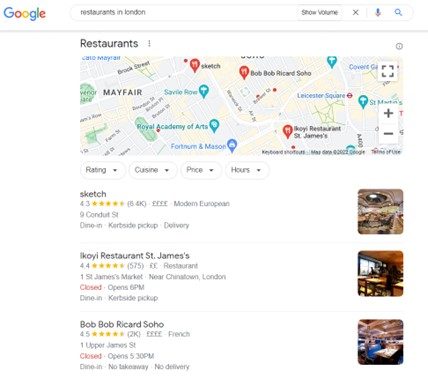This Google search results screenshot captures a detailed view of the webpage layout for the query "restaurants in London." The header stands out with its clean white background, featuring the multicolored Google logo on the left-hand side. Adjacent to the logo is a white search bar with rounded ends and a thin, medium-gray outline. The search bar contains the black typed text "restaurants in London," followed by a small gap, leading to a white rectangle bordered by a light gray outline. Inside the rectangle, black text reads "show volume." Further to the right, the search bar includes a dark gray 'X' icon, a vertical light gray separator line, a multicolored microphone icon, and a blue magnifying glass icon, all contributing to the search functionalities.

Underneath the header, a medium-gray shadow casts onto the main body of the webpage, which is white. At the top-left corner of the body, the black bold text "restaurants" is prominently displayed. To its right, three medium gray dots are aligned vertically, while the upper right corner hosts a dark gray eye icon surrounded by a dark gray outlined circle, indicating additional viewing options or settings.

Below this section, a wide, landscape-oriented map captures attention. The map showcases beige and gray land areas intersected by curving white roads, some marked with dark gray arrows. Various pins in teal, medium blue, and red punctuate the map, each containing different white icons and corresponding color-coded text, except for the red pins which are paired with black text annotations. 

At the bottom of the map, four pill-shaped buttons offer filtering options, each adorned with dark gray text: "Rating," "Cuisine," "Price," and "Hours." These buttons have a white fill and light gray thin outlines, with a dark gray downward-pointing triangle next to the text, signaling drop-down menus for further refinement of search results.